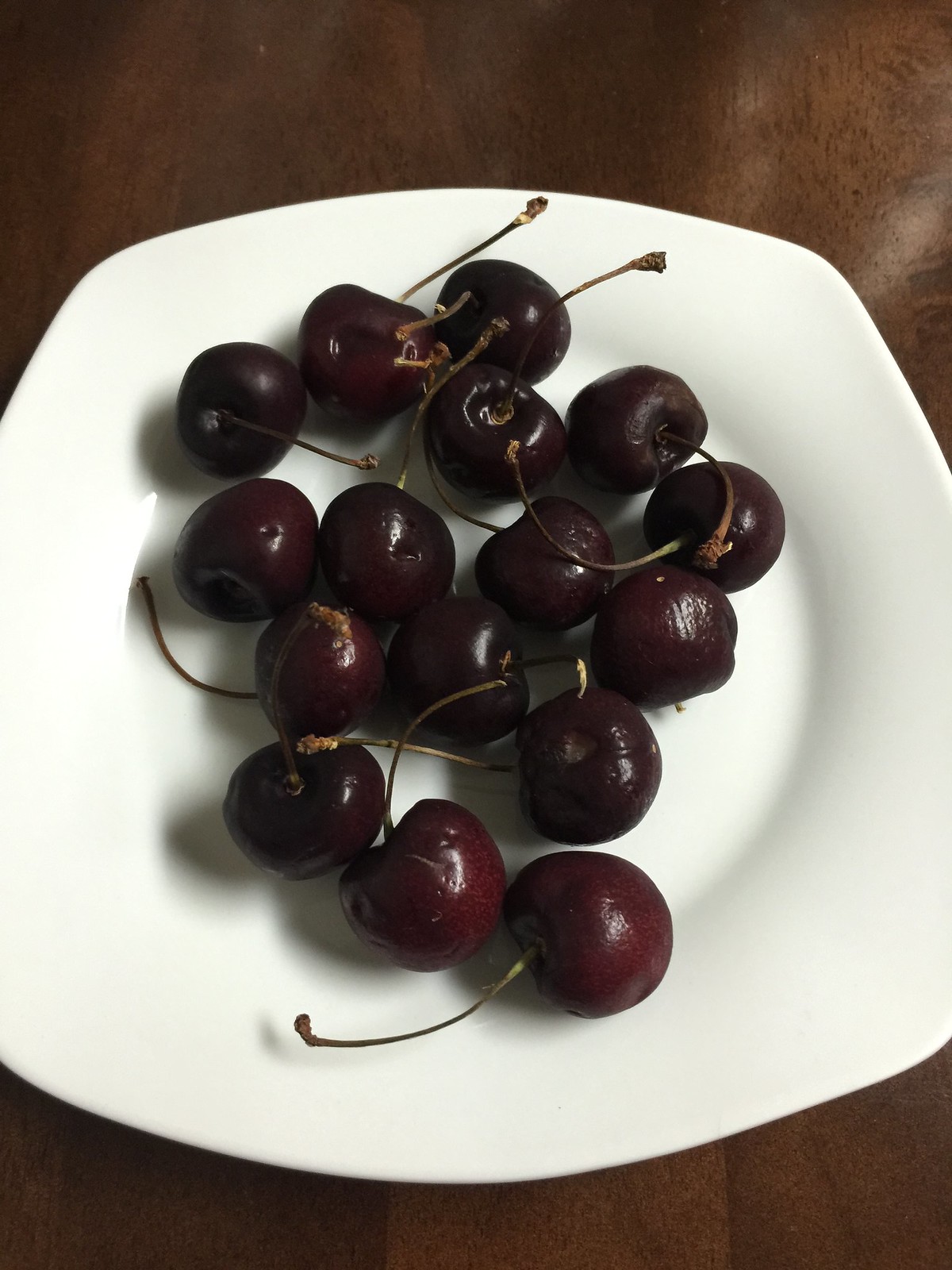In the photograph, a white, slightly oval plate is centered on a dark brown, polished, wooden table. The plate holds approximately 15-17 cherries, each with stems still attached, fanning out in various directions. The cherries are a deep, dark red color, indicating they have just been picked, though some exhibit slight wrinkling. This gives a sense of natural imperfection. The cherries are randomly distributed, covering most of the surface of the plate. The background features a subtle glimpse of brownish fabric, adding texture to the setting.